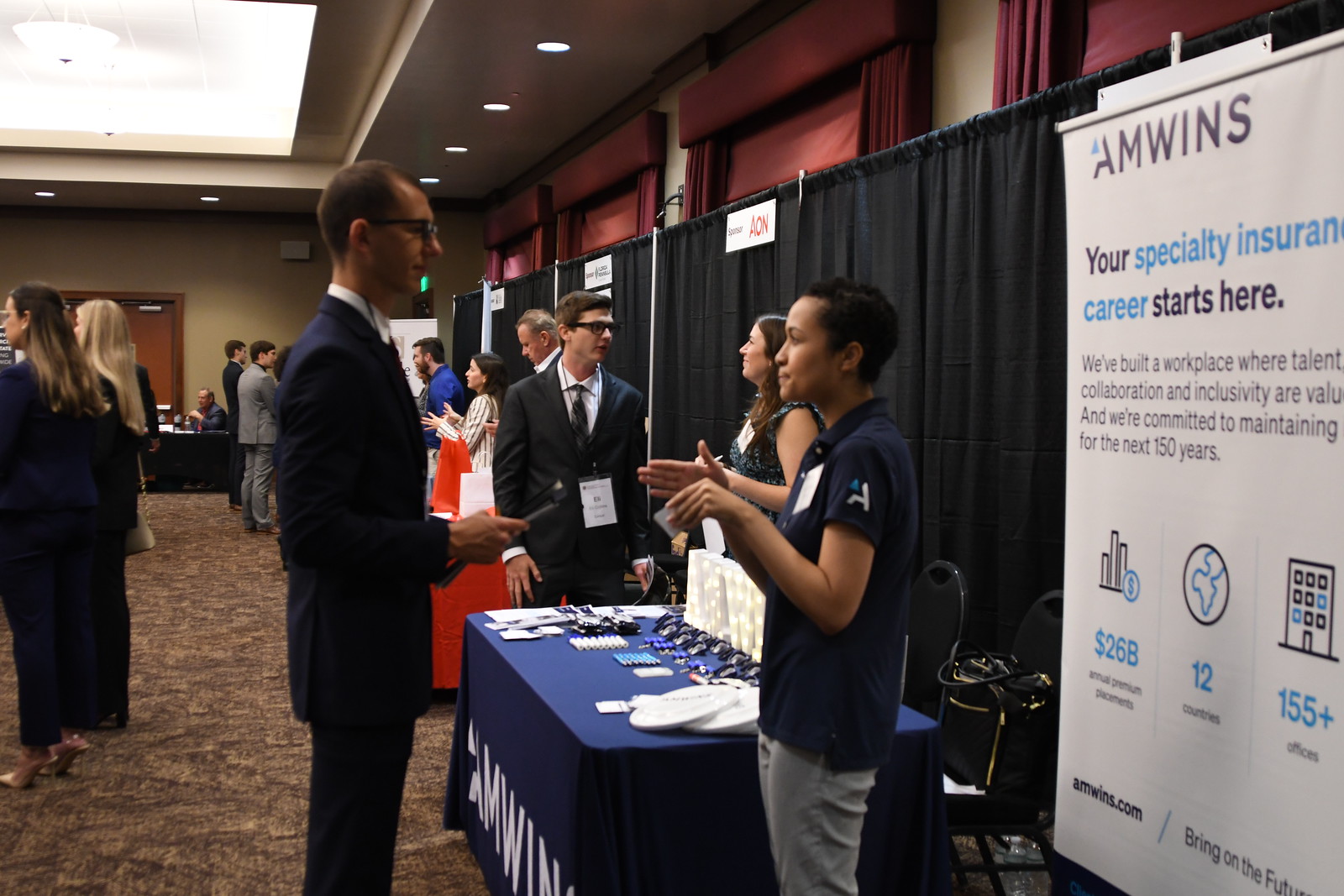The image captures a lively scene at a job fair or conference. On the right side, there is a long, black partition curtain that creates a makeshift wall. In the foreground, a blue folding table is adorned with various items and features a banner that prominently reads, "Your specialty insurance career starts here." Text is visible beneath this slogan, suggesting detailed information about career opportunities. 

At the table, a man in a dark blue suit, white shirt, and glasses is engaged in conversation with a woman wearing a blue polo and gray slacks. She has very short hair and appears to be of Asian descent, possibly Filipino. In the background, more formally dressed individuals can be seen milling around, indicative of a bustling networking event. The venue has brown carpeting and a white ceiling studded with lights, creating a bright environment. Additional details include the presence of doors in the distance and the name "AmWins" displayed prominently on the banner and tablecloth. The atmosphere exudes a professional and engaging event focused on career building within the insurance industry.